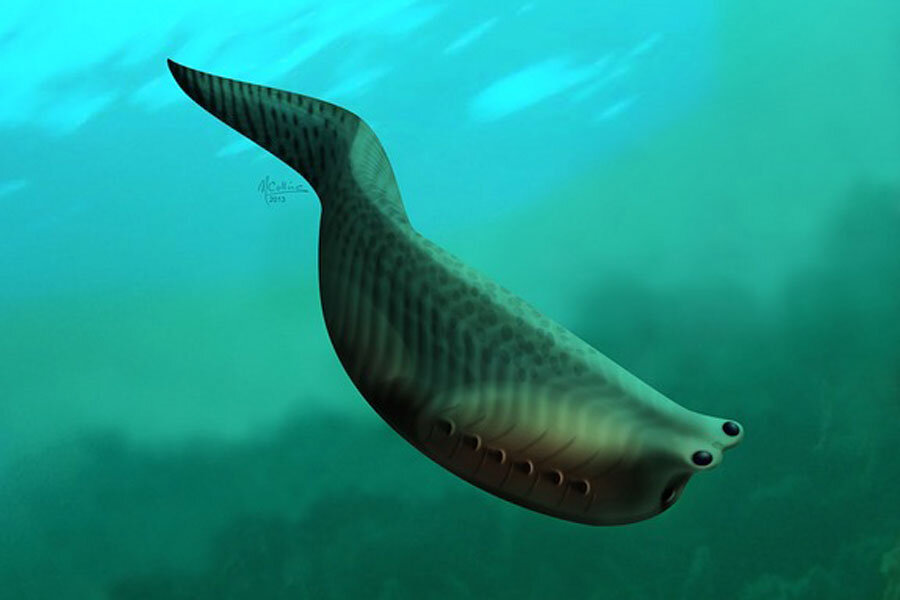The artwork portrays an underwater sea creature against a turquoise ocean backdrop with various murky details suggesting the seabed. Signed by the artist in small black handwriting to the left of the creature, the digital illustration—a blend of blues and greens—depicts a unique, fantastical being resembling a hybrid of an eel, fish, and sea slug. The creature is oriented diagonally, with its bulkier head pointing toward the bottom right and tapering tail extending to the top left. Its body, covered in a variegated gray and bluish-green scaly pattern with black striations, features noticeable yet mysterious attributes: six circular breathing holes on each side near its head and two prominent black eyes protruding from atop its head. The setting emphasizes this marine anomaly amidst a murky, sunlight-pierced ocean, dotted with aquatic plants in the subdued greenish-brown water below.